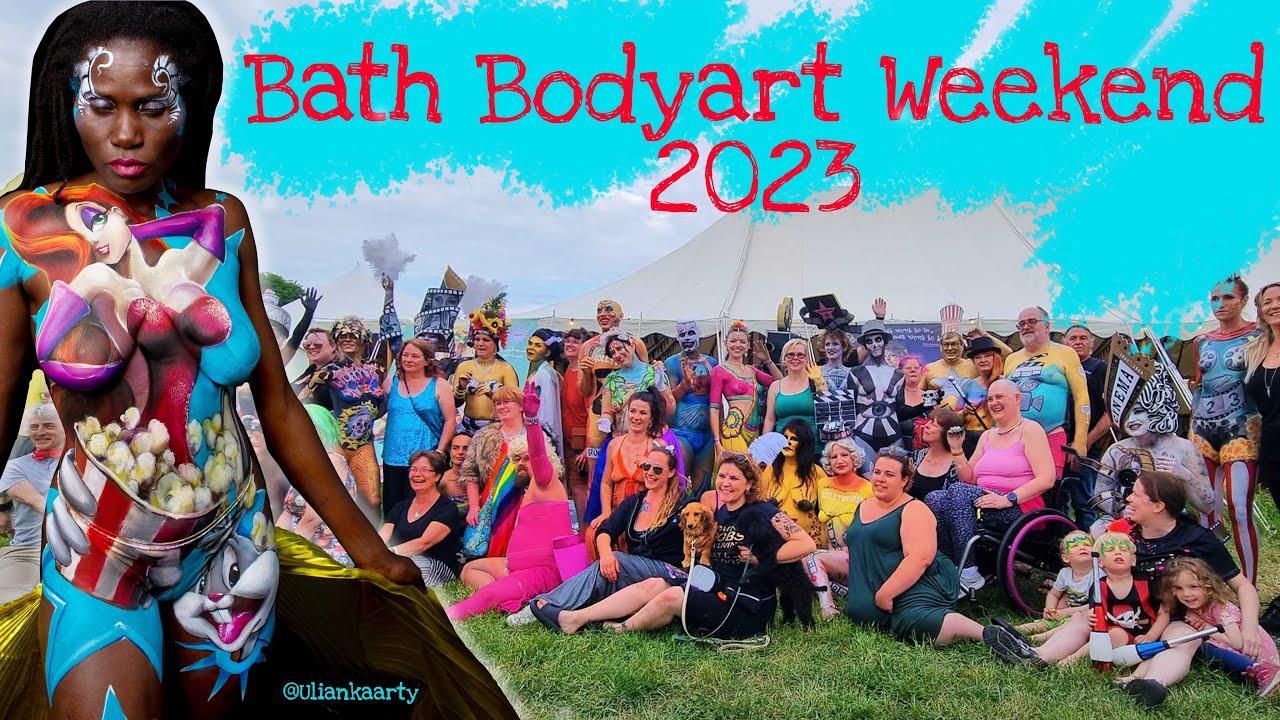The photograph is a vibrant, detailed scene from Bath Body Art Weekend 2023, as indicated by red text at the top against a teal, spray-painted background. In the foreground, a striking dark-skinned African-American woman, standing left and slightly superimposed over the main scene, captures immediate attention. Her long, straight hair is combed back, and she's adorned in elaborate body paint, featuring Jessica Rabbit emblazoned across her chest, and Bugs Bunny on her left leg. Her chest and waist also showcase a retro-style popcorn carton with red and white stripes, accompanied by white flourishes around her temples and purple eyeshadow framing her eyes. 

Next to her, an array of people are seated and standing on a grassy green field, their bodies adorned with diverse body paints. Children are positioned in the front, next to several individuals in wheelchairs. One notable participant, a woman on the far right, has a film strip painted on her belly, indicating "two" and "three," with blue and red striped legs. The backdrop of the image is a serene turquoise sky dotted with white clouds, enhancing the lively and artistic atmosphere of the event.